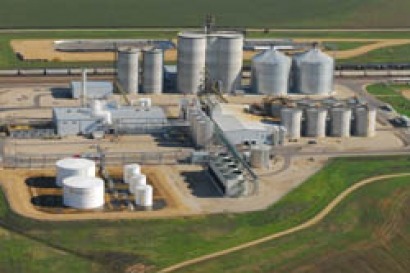The image is a slightly angled aerial view of a large industrial farm complex surrounded by expansive, flat grassland. The photograph showcases a variety of cylindrical structures and metal buildings typically used for storage and processing. In the foreground, there are two large white cylinders that resemble gasoline storage tanks and three smaller white tanks situated to their right. Dominating the middle ground are numerous silver metal structures, including tall, cylindrical towers that suggest storage for liquids, grain, or silage. Notably, in the background, there are six large silos with different shapes—two smaller ones on the left, two very large ones in the center, and two slightly shorter but broader ones on the right, which interestingly have lids resembling cookie jar tops. The plant complex is primarily composed of single-story, aluminum-colored buildings with flat roofs. Surrounding the buildings is a network of dirt or gravel roads and possibly a railroad line that integrates into the industrial area. The scene also features a gray building, likely used for operations, and notable tracks indicating where farm machinery, such as tractors, has traversed, highlighting the facility’s heavy integration with the surrounding agricultural fields.